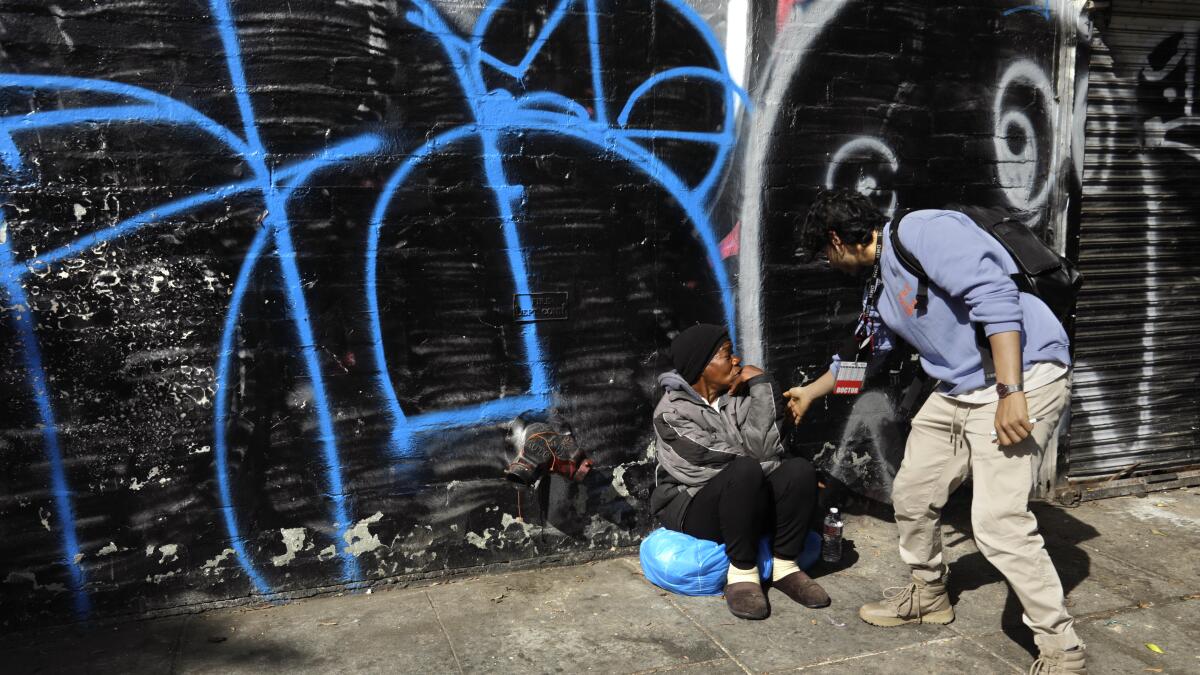In this photograph, taken outdoors on a sunny day with sunlight casting shadows on the surroundings, we see an emotionally charged interaction between two individuals on a concrete pedestrian walkway. The backdrop features a black cinder block wall adorned with blue and white graffiti, alongside a black rolling shutter door also covered in graffiti. Standing on the right, one person, possibly a young man, wears tan-colored boots, gray sweatpants, a blue long-sleeve sweatshirt with sleeves rolled up to the elbows, and a black backpack. He's gently patting the shoulder of a man sitting on a crumpled blue trash bag. The seated individual, who appears to be homeless, is dressed in brown slippers with white socks, black sweatpants, and a gray and black hoodie. His head, covered by a black hood, rests on his hand as he looks away, seemingly indifferent to the interaction. The detailed attire and positions of the two create a poignant scene, highlighting the social disparity and compassionate outreach taking place.